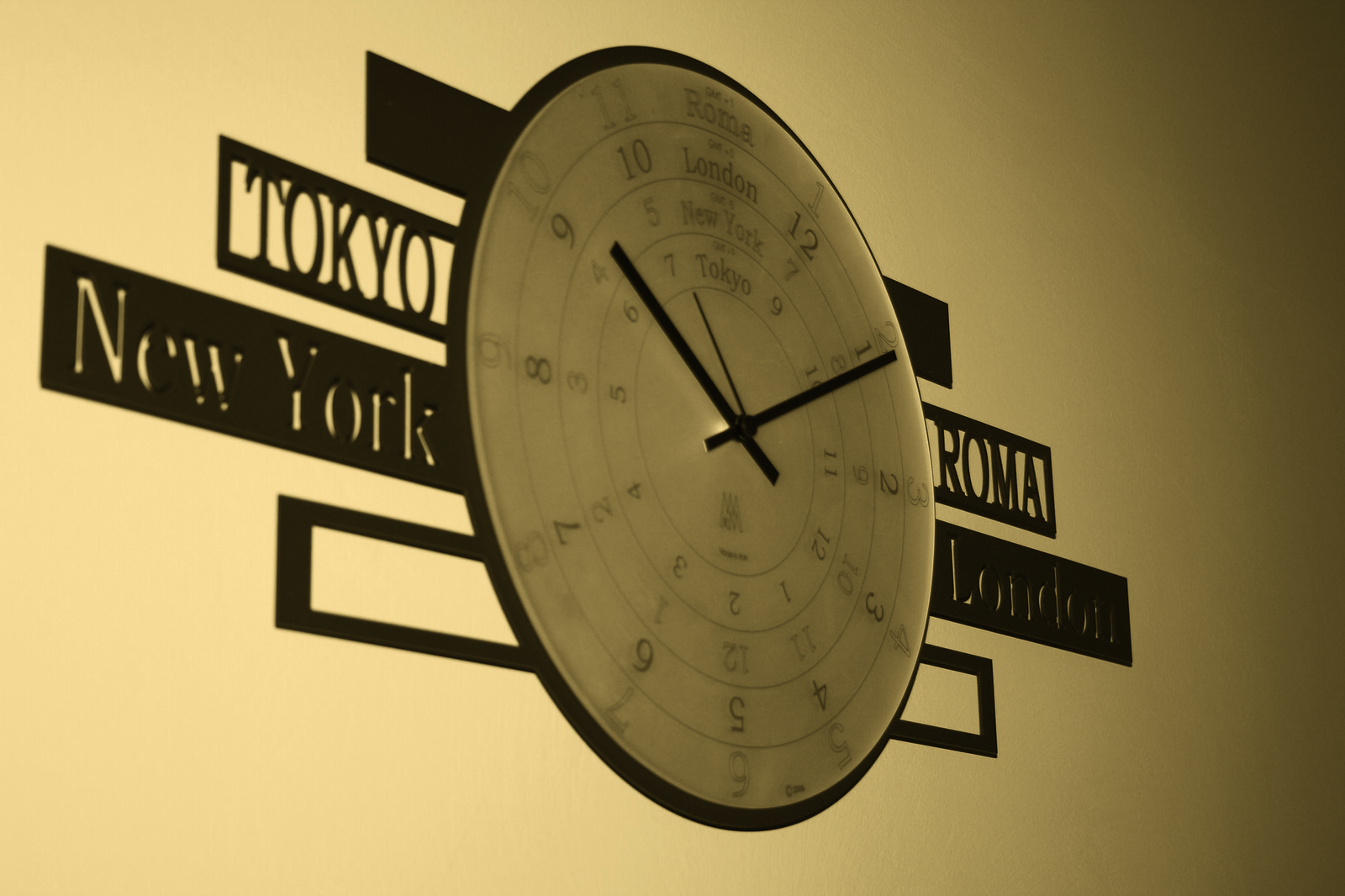This is a photograph of a unique, multi-timezone clock mounted on a pale yellow wall. The clock face is circular and white, outlined in black, and features four concentric circles to indicate the time in four different cities: Tokyo, New York, London, and Rome. The innermost circle displays Tokyo's time, followed by New York, then London, and the outermost circle shows Rome. The clock has dark-colored numbers and hands, including a second hand. Labelings for each city—"Tokyo," "New York," "London," and "Roma"—are engraved in dark letters on the clock face.

The background behind the clock is divided into several brown rectangular sections with intricate details. The top section has a solid brown rectangle, and below that is a brown rectangle with metal letters that have cut-out centers allowing the yellow wall to show through. To the left of the clock, the word "Tokyo" is visible, and to the right, it says "Roma." A longer brown rectangle beneath these labels displays "New York" on the left, with the cut-out centers showing the wall behind, and "London" in raised dark lettering on the right. At the bottom, there's an outline of a thick brown rectangle with an open center. The entire setup creates a surrealist aesthetic with a functional purpose, showcasing the time in four major world cities simultaneously.